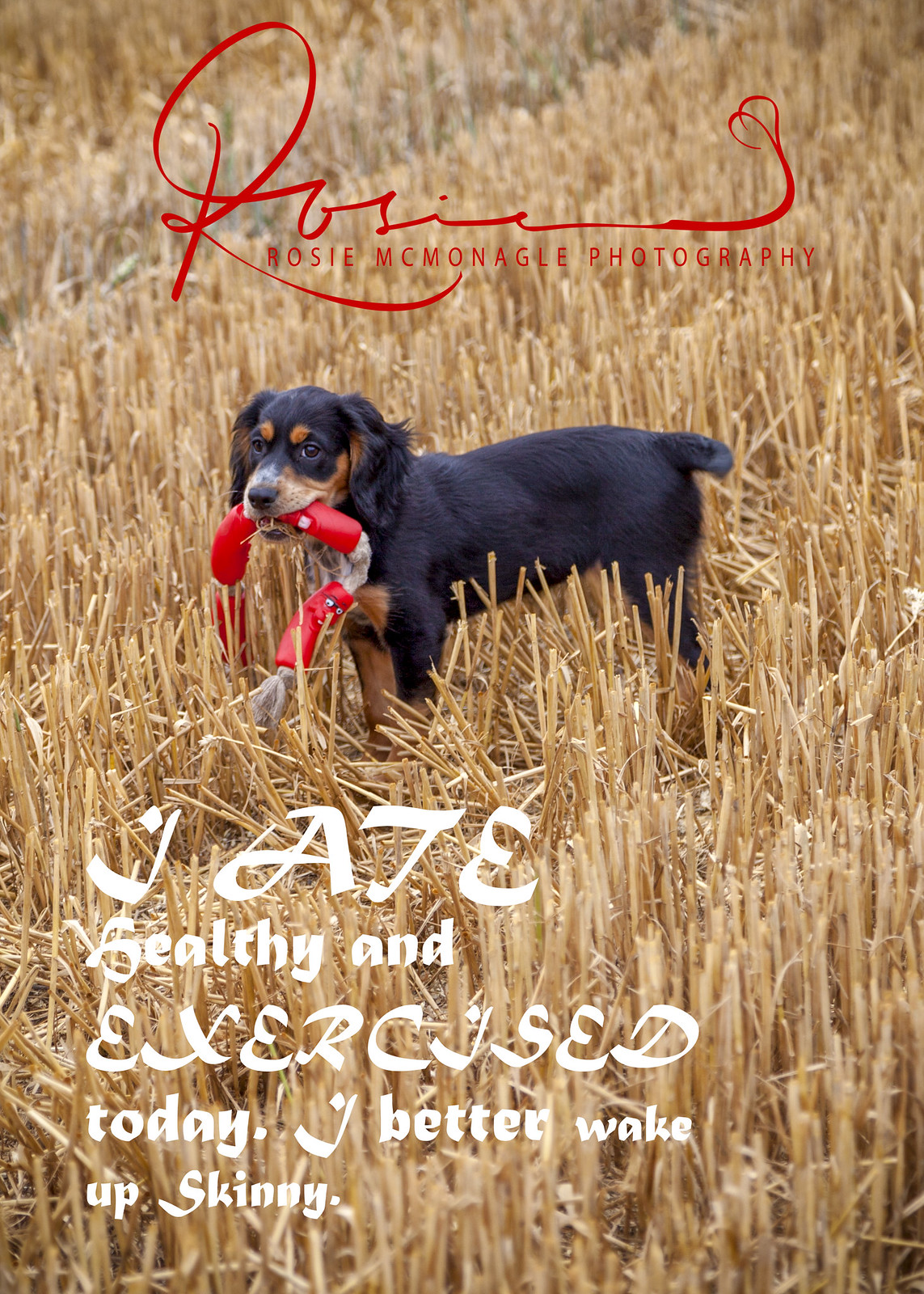The image features a black Spaniel puppy with tan markings on its chest, around its eyes, and underneath its ears, as well as a white-tipped muzzle and a black nose. The puppy, which is being trained for hunting exercises, stands in a field of freshly cut straw or hay with tall, sturdy yellow stalks everywhere. It is holding a white rope with three or four red rubber sections interspersed within the rope, possibly squeaky toys. At the top of the image, in red cursive with a large, flourished "R," is the signature "Rosie." Below it, in red print, is "Mosey-McMonigle Photography" or variations such as "Rosie Mimungle" or "Rosie McMonagle Photography." Underneath the puppy, in white stylized lettering with changing font sizes, reads the playful caption: "I ate healthy and exercised today. I better wake up skinny." The photograph, taken outdoors in portrait mode, advertises the photography studio while showcasing the puppy amid the golden field under the bright daylight.